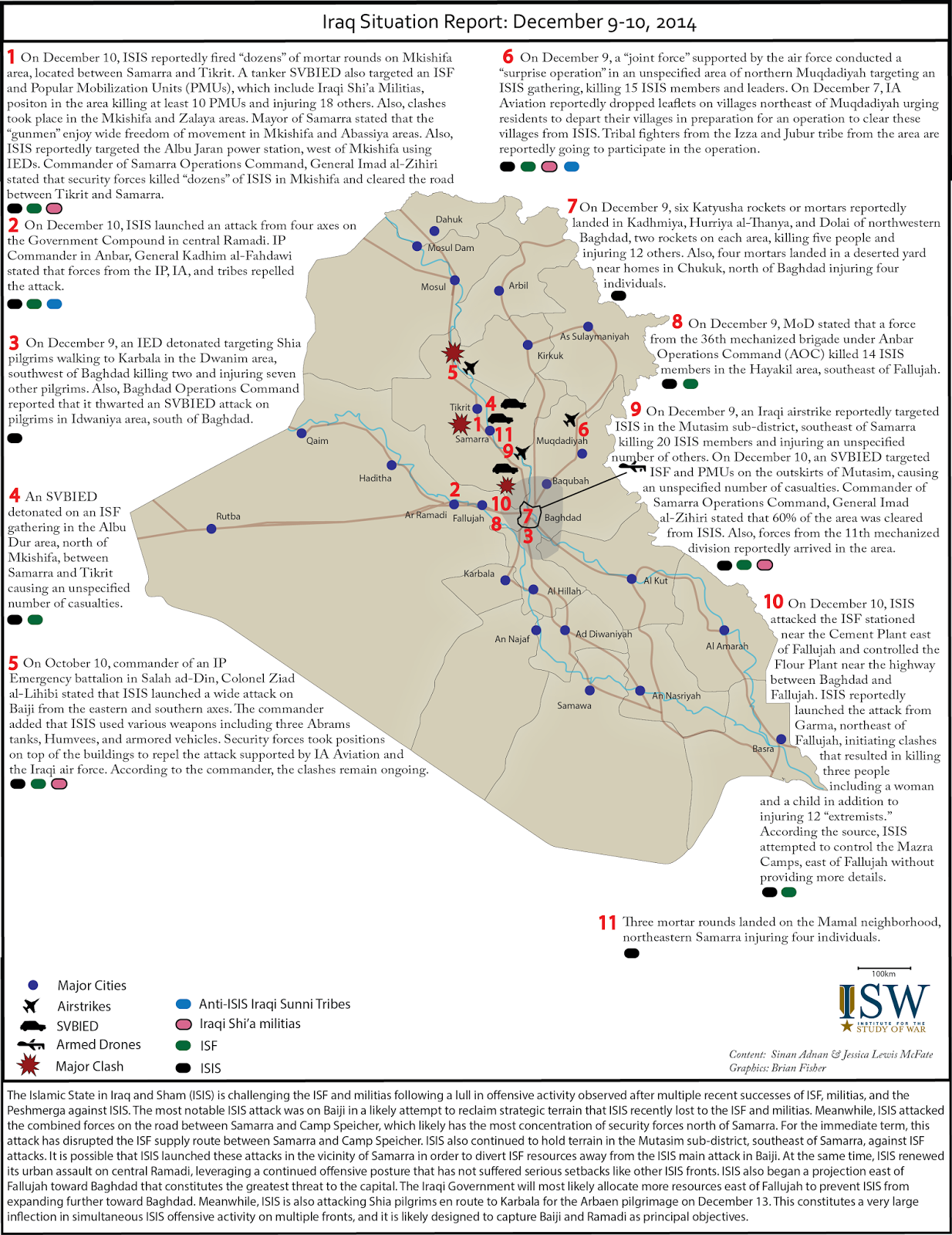Detailed Caption: 

This image showcases a comprehensive news report titled "Iraq Situation Report" covering events from December 9th and 10th, 2014. The report is densely packed with information, featuring 11 distinct points each marked with red numbers from 1 to 11. Each point is detailed in black text, with the content being relatively small in size. Notably, the 1st point details an incident from December 10th, where ISIS reportedly fired several mortar rounds in the area between Samarra and Tikrit.

In the center of the report, there is a detailed map of Iraq with various cities and regions marked by lines. The map itself is numerically coded to correspond with the key points detailed in the report. Surrounding the map, there are color-coded keys that are crucial for interpretation: black, green, and pink bubbles, each representing different entities—ISIS, the Iraqi Security Forces (ISF), and Iraqi side leaders, respectively.

At the bottom of the report, there is a disclaimer section providing additional context or information related to the report, along with a mention of "SW," indicating the publisher or the organization responsible for the report. The combination of text, map, and color-coded keys provides a thorough visual and textual analysis of the situation in Iraq during the specified dates.